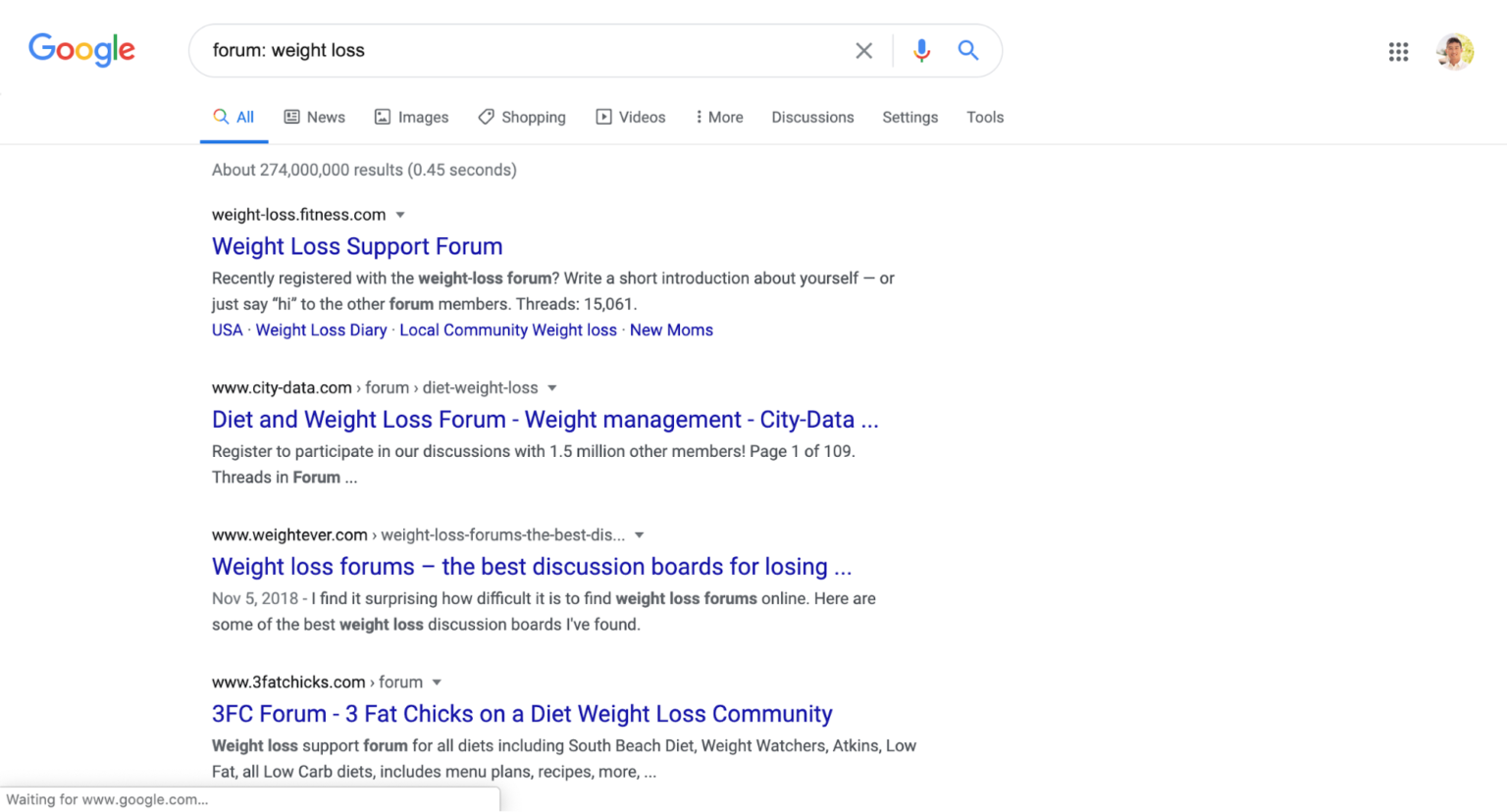A screenshot captures a Google search results page. The search query entered is "Forum Weight Loss." Below the search bar, the results indicate approximately 274 million hits. The first result is for weightloss.fitness.com, titled "Weight Loss Support Forum." The second result points to www.city-data.com/forum/diet-weight-loss, with the title "Diet and Weight Loss Forum, Weight Management City Data." The third link, www.weightever.com/weight-loss-forums-the-best-dls, is labeled "Weight Loss Forums: The Best Discussion Board for Losing." The final search result listed is www.3fatchicks.com/forum, titled "3FC Forum - 3 Fat Chicks on a Diet Weight Loss Community." Each link suggests various online forums dedicated to weight loss, offering support, discussion, and resources for individuals seeking weight management advice.